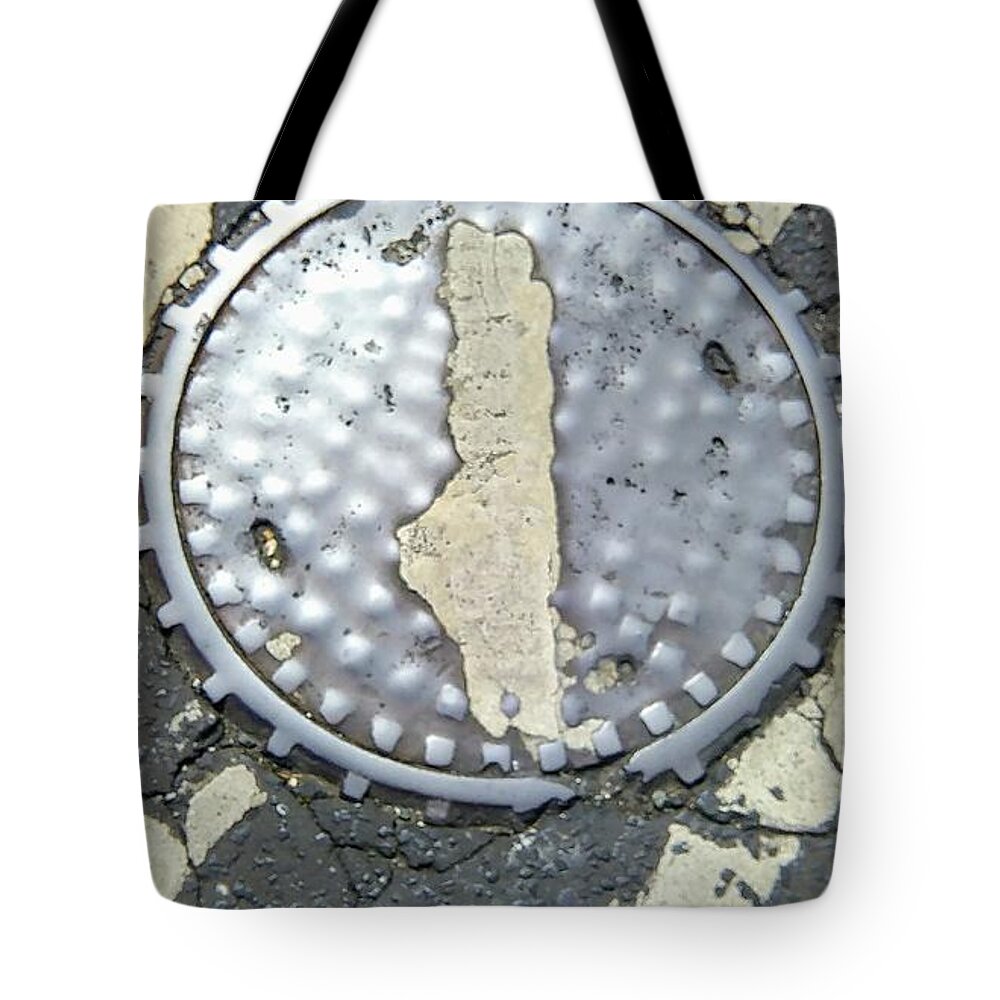The close-up image portrays an intricate piece of steampunk and industrial-inspired art, featuring a well-worn, silver manhole cover that has been painted over and reset at an off-kilter angle. This manhole cover, full of character with its battered knobs and worn-out surface, forms the central element of the artwork. It rests upon a rugged, concrete-like substance that displays varying shades of white and dark gray, suggesting areas of wear and resurfacing. The edges of the concrete mimic the texture of aged asphalt, further framing the manhole cover. The entire piece is suspended on a black ribbon, adding an industrial aesthetic to its presentation. This unique artistry, captured on what appears to be a canvas bag, combines the raw textures of metal and concrete, evoking a sense of urban decay and resilience. The juxtaposition of the manhole cover with the surrounding, broken blacktop pattern, accentuated by the misaligned road stripe, enhances its visual impact, making it a compelling focal point for the viewer.